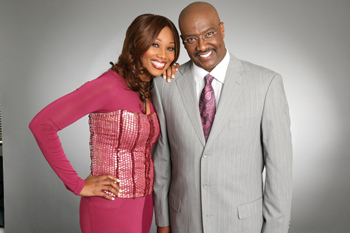The photograph features two middle-aged, African American individuals posed and smiling directly at the camera. They appear to be professionals, possibly actors or news broadcasters. The background behind them transitions from a light gray in the center to a darker gray and edges into black towards the corners. The woman on the left is dressed in a long sleeve pink dress with her torso embellished by a sequined tube top. She has shoulder-length brown hair, her left hand is resting on the man's shoulder while her right hand is placed on her hip. The man to the right, who she is leaning on, has a bald head, glasses, and a mustache reminiscent of Steve Harvey. He is dressed in a gray business coat with a white button-up shirt and a pinkish-purple maroon tie. Both individuals exude a sense of charm and sophistication, sharing a warm smile with the viewer.